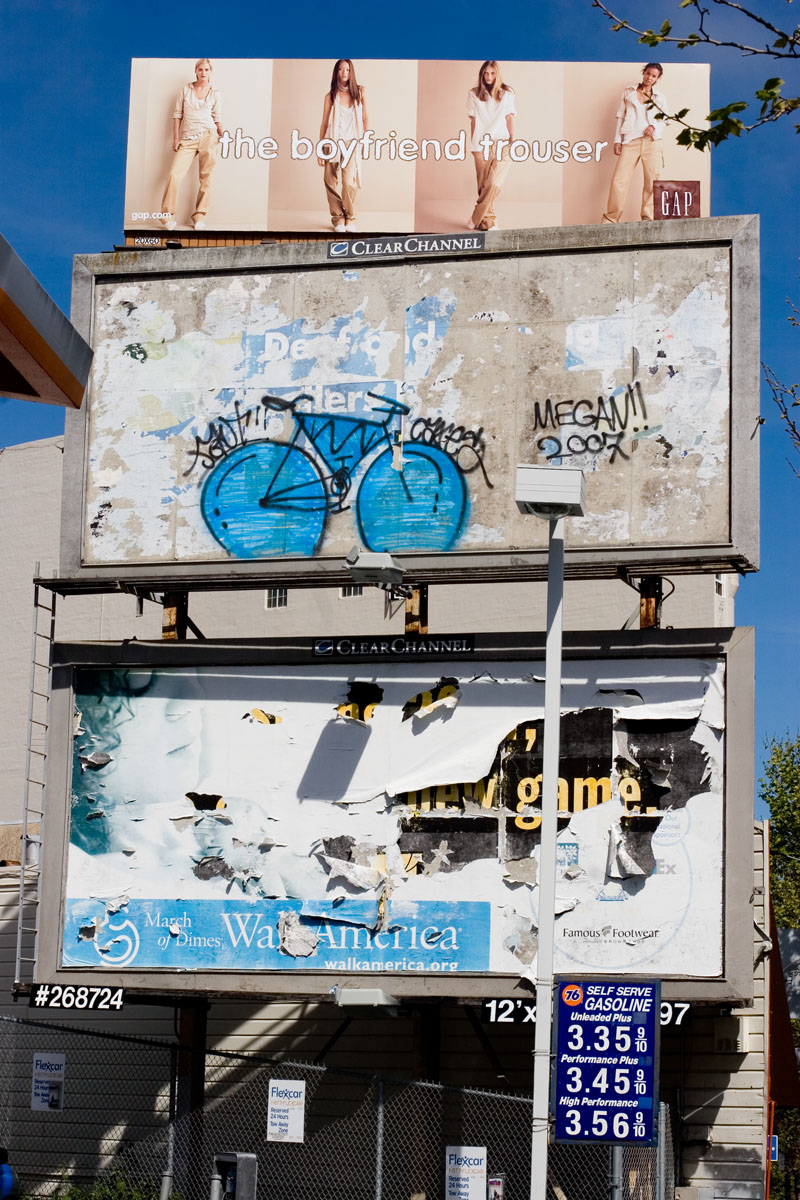The image showcases a set of three billboards, set against a clear blue sky with scattered trees. The most prominent billboard at the top features an advertisement for GAP, promoting "The Boyfriend Trouser." This billboard presents four women modeling the trousers, paired with white shirts, with the brand's logo visible in the bottom right corner. 

Below it, the middle billboard is heavily worn and largely obscured by graffiti, including a prominent blue bicycle and the tag "Megan 2007." This billboard has faded to the point where its original message is no longer discernible. 

The bottom billboard is similarly eroded, partially revealing an advertisement for the March of Dimes' "Wall America." This sign is almost completely deteriorated, with remnants of the text barely visible. 

In the foreground, a lamppost holds a blue sign indicating prices for self-serve gasoline, listed as $3.35, $3.45, and $3.56. 

A grayish-white building and a fence are visible behind the billboards, with the brand name "Clear Channel" noted at the top, likely identifying the company responsible for the advertisements. The scene captures a vivid juxtaposition of commercial advertisement decay against a backdrop of urban elements and nature.